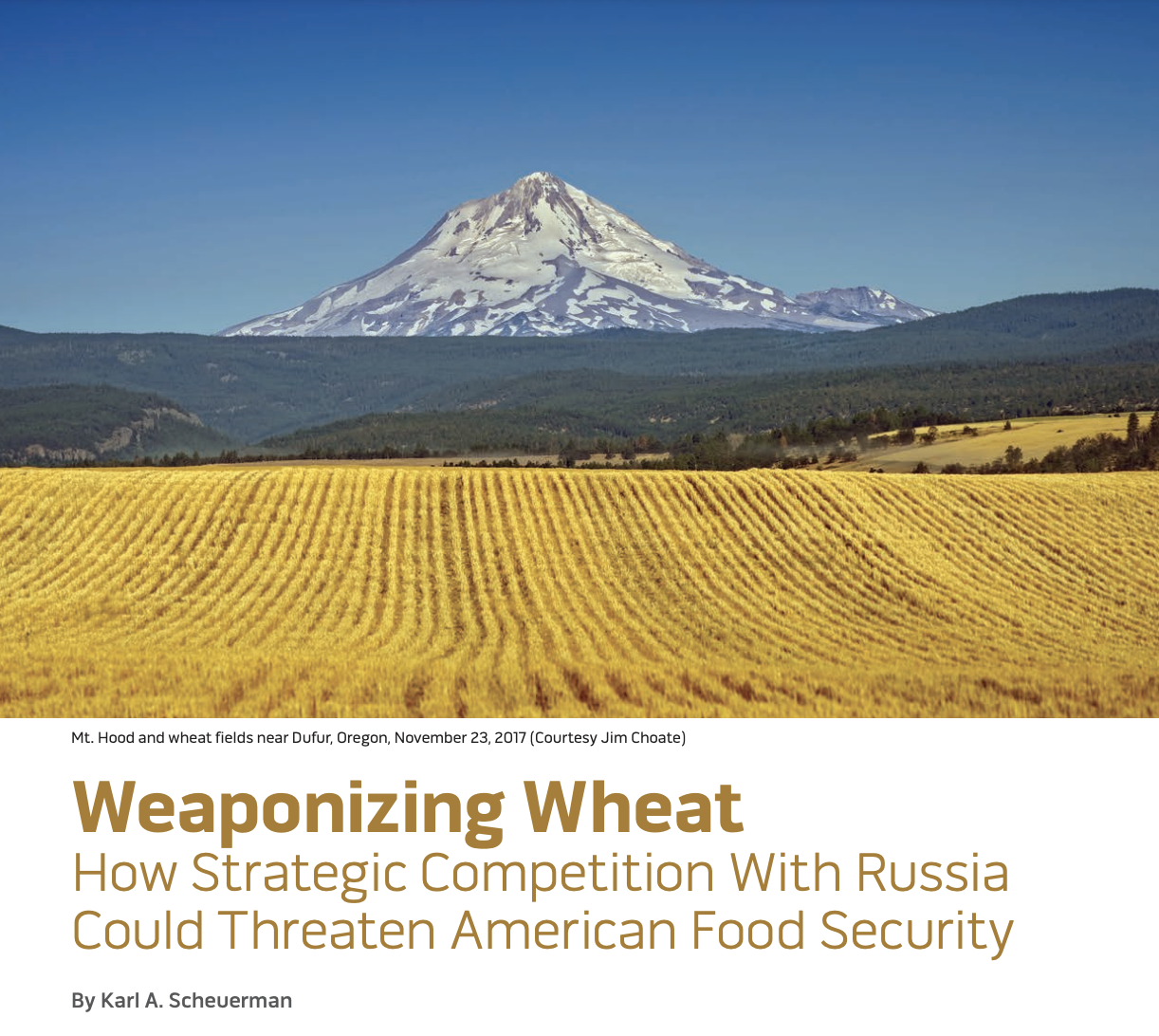Mount Hood and Wheatfields near Dufur, Oregon, November 23, 2017 (Courtesy of Jim Choate)

The hero image at the top of this article showcases a stunning landscape featuring Mount Hood in the background, its rugged peaks blanketed with snow and a grayish tint. Below lies a lush green forest, extending into golden-yellow wheat fields with splotches of brown in the foreground. The sky above is a gradient of blue and cyan, lending a clear, daytime atmosphere to the scene. This picturesque photograph exudes the serene beauty of the Oregon countryside. 

Beneath the image, the text reads:
"Weaponizing Wheat: How Strategic Competition with Russia Could Threaten American Food Security" by Carl A. Schuerman. The caption, title, subtitle, and credit line are presented on a white background, with the caption and byline in black text, and the title and subtitle in a brownish wheat-colored font.